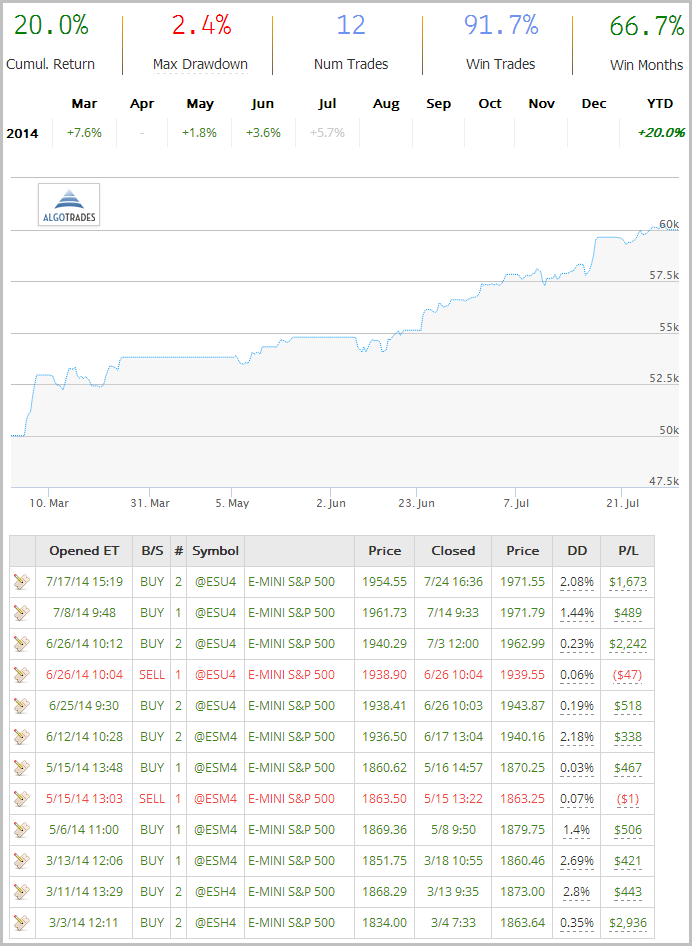The image primarily depicts a detailed financial report that incorporates a variety of metrics and statistical data presented in multiple segments.

At the top of the image, there is a collection of numbers mainly represented as percentages, displayed horizontally from left to right. These numbers include:

- 20.0% in green, labeled as "Cumul." (presumably short for Cumulative Return), accompanied by a yellowish-black bar beside it.
- 2.4% in red, labeled as "Max Draw Down," with a similar colored bar to its right.
- The number 12 in blue, followed by the term "Num Trades" in black, along with its corresponding bar.
- 91.7% in light blue or purple, noted as "Win Trades," with a matching bar next to it.
- 66.7% in green, marked as "Win Months," accompanied by an equivalent bar.

Below this, a series of monthly abbreviations (MAR, APR, MAY, JUNE, JUL, AUG, SEP, OCT, NOV, DEC) and the acronym YTD (Year To Date) are listed in black letters. Underneath these abbreviations, and specifically for the year 2014, the report shows monthly performance data with green positive percentages for certain months: 
- March (+7.6%)
- May (+1.8%)
- June (+3.6%)
- July (+5.7%)

Other months are left blank, symbolizing no data.

Under this section is an extensive gray bar, followed by a small, boxed emblem in gray and blue formatting of an upward-pointing triangle with varying shaded lines. Beneath this, the text "Blue Algo Trades" appears prominently.

Further down, the image showcases a faint graph plotted on a grid marked with numerical scales ranging from 60K to 47.5K on the right. A prominent blue line weaves through the graph starting low and trending upwards, with the area below the graph shaded in faint purple. Dates are along the bottom (10Mar, 31Mar, 5May, 2June, 23June, 7JUL, 21JUL), which likely signify the tracking periods of the company's stock performance over several months. The assumed stock "algo trades" may refer to algorithmic trades.

At the base of the report, there is a large table-like structure packed with a variety of statistics. The table includes a key across the top defining different categories: "OpenDT," "B/S," "#," "Symbol," "Price," "Closed Price," "D," "P/L," each separated by faint gray lines.

The table is a comprehensive record of trading activity, showing:
- A possible logo resembling a newspaper and pencil.
- Dates and times (in red or green) for buying or selling actions.
- Symbols like E-S-U-4 and specific stock tickers.
- Prices in a detailed numerical format (e.g., 1971.55).
- Closing dates and times in military format (e.g., 7-24, 1636).
- Various percentages under categories labeled D and P/L in black, green, or red.

This financial report ultimately offers an extensive summary of algorithmic trading results, performance metrics, and detailed transaction records, reflecting thorough data capturing and analytical clarity.